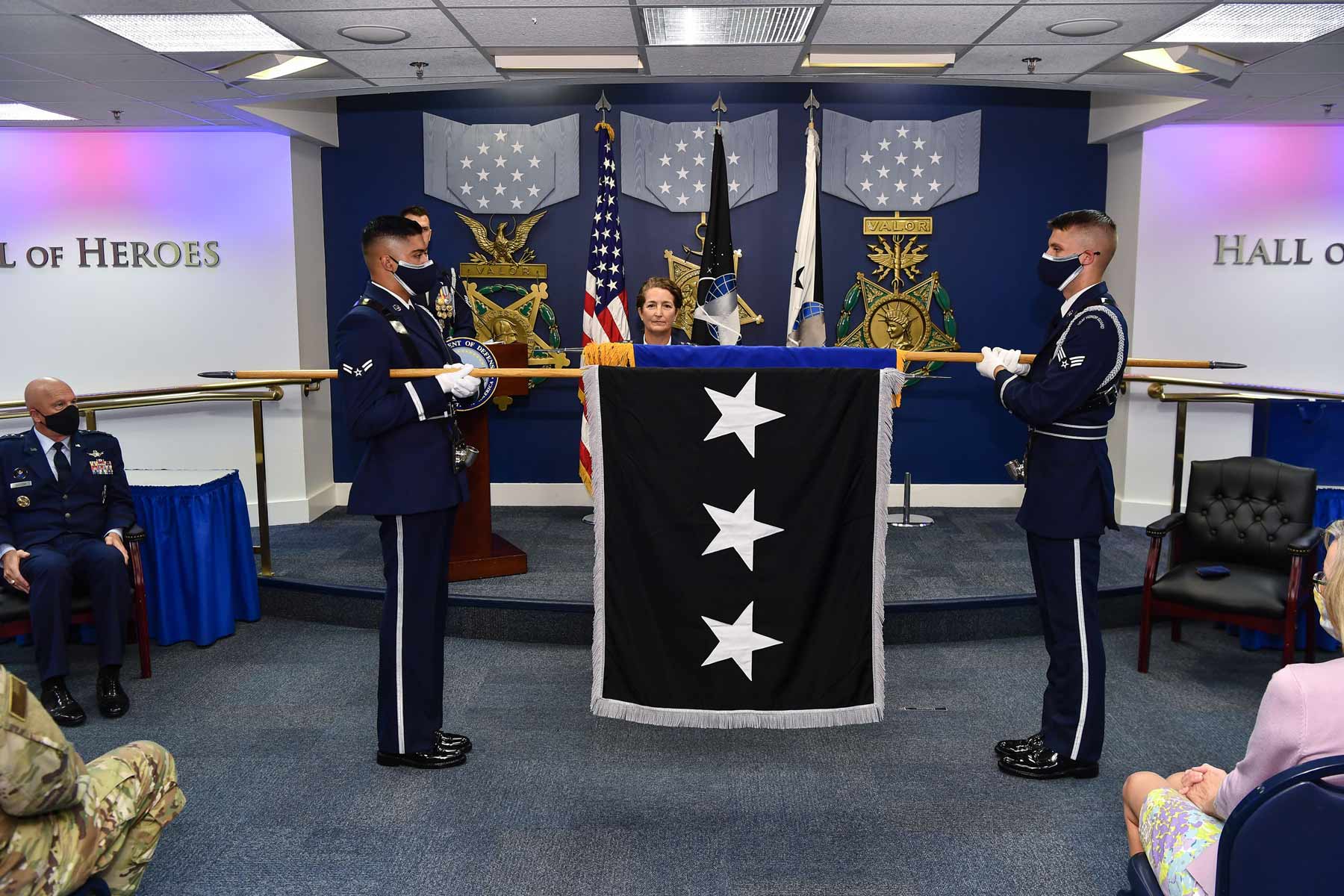The image depicts an indoor military ceremony set in a room with white walls labeled "Hall of Heroes" in silver lettering on either side of a central podium. Behind the podium stands a woman, and flanking her are two large shields and an American flag. In front of her, two servicemen in military uniforms and masks are holding a black flag with three white stars. Another masked serviceman is positioned to their left, and another individual in camouflage can be seen in the corner. The ground is covered in blue carpeting. The room features additional seating for attendees, including a woman in a skirt seated to the right. The ceremony appears to involve flag handling, as the two servicemen are either rolling up or unrolling the flag. The background also displays three large military medals, adding to the solemn and formal atmosphere of the ceremony.